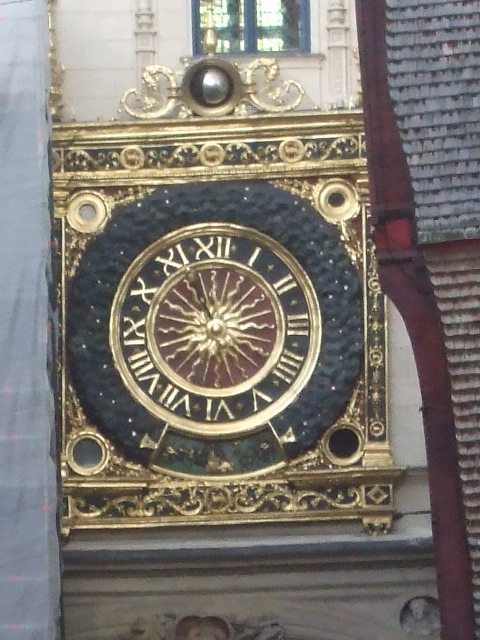This is an image of an antique-style, large, gold metal clock mounted on the exterior of a beige building. The clock, which features a sunburst design radiating from the center, has black Roman numerals on a gold-outlined black face. The gold clock hands rest over a black circle in the middle of the sunburst. Surrounding this circle are four decorative gold holes that appear black inside, with intricate gold scroll designs and round gold accents on top. The building, trimmed in black, has a portion of its brown wooden paneling visible below the clock. A purple-burgundy stripe runs vertically down the building, adding a splash of color. Above the clock is a stained-glass window in shades of blue and green, highlighted with white to mimic light reflection. To the right of the clock, there is a section reminiscent of roof shingles, and further down, there's a gray area that might be another part of the building. The architectural elements include etchings and accents, giving the structure a vintage and decorative appearance.